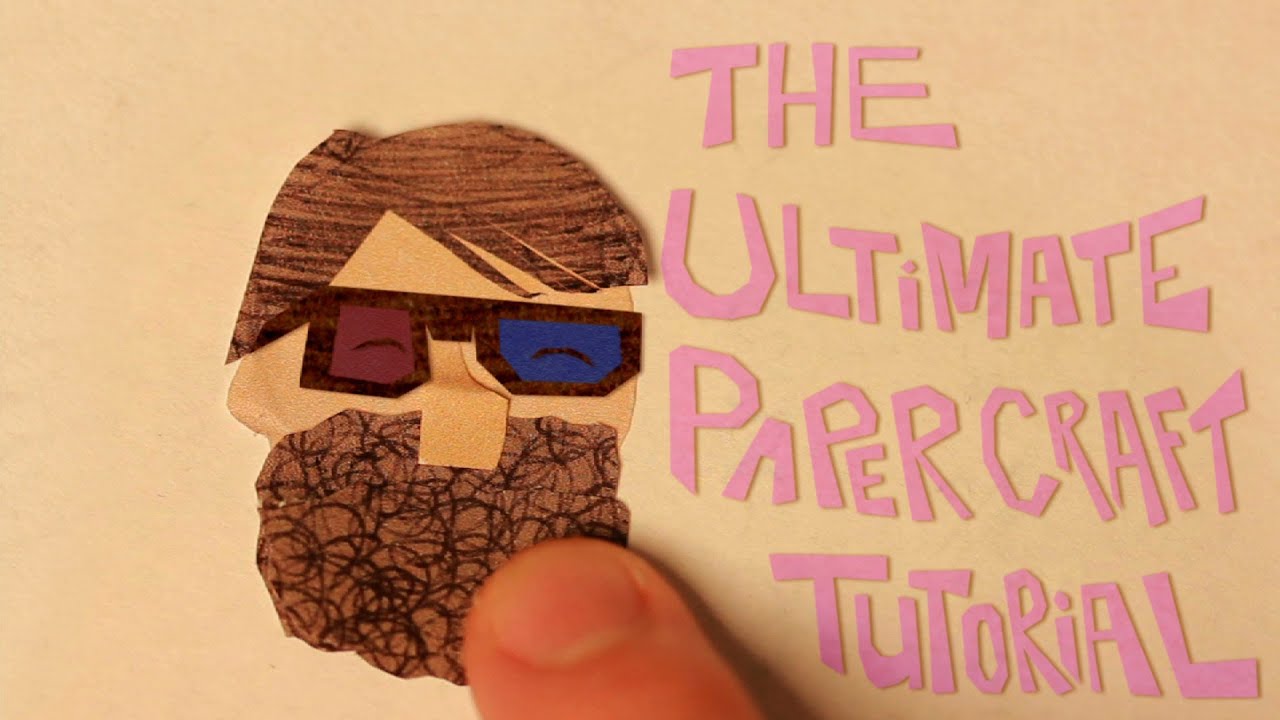In the image, there is a meticulously crafted papercraft artwork set against a tan-colored background. Dominating the left side of the image is the face of a man made entirely from paper. The man features brown hair and a large, curly brown beard. His eyes are represented as squinted lines, and he wears a pair of black-framed 3D glasses, with the right lens colored blue and the left lens red. No visible mouth is included in the design. To the right side of the man's face, in large pink paper letters, the words "THE ULTIMATE PAPERCRAFT TUTORIAL" are displayed, each word stacked on top of the other in four lines, and all letters are capitalized. At the bottom of the image, slightly overlapping the beard, a human thumb—belonging to a Caucasian individual—presses down gently on the paper beard, adding a tactile element to the visual.